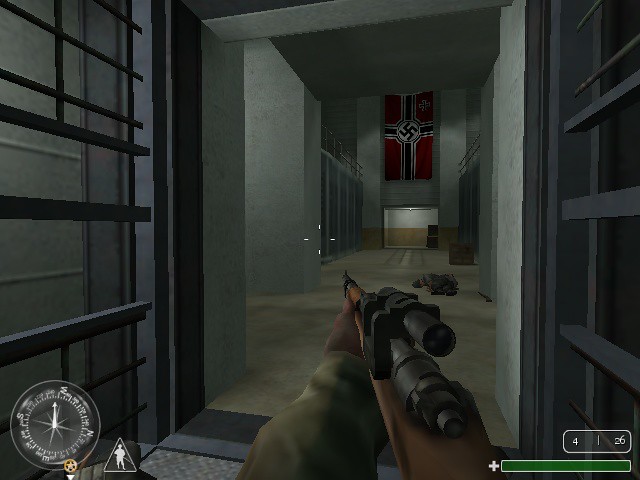The image captures a detailed screenshot from a first-person shooter video game. The setting is a stark, gray-walled room, likely constructed of concrete or stone, giving a cold, militaristic feel. The viewer’s perspective is from a first-person viewpoint, with the foreground dominated by the top of a gray rifle, held by hands clad in a camouflage uniform, and visible sights indicating aim. Flanking the walkway are barred windows, reinforcing the sense of enclosure.

In the center of the room, slightly blurred but recognizable, lies a dog next to a fallen figure sprawled on the gray floor, with a black gun laying adjacent. This scene suggests a recent combat scenario. Prominently mounted on the back wall is a large, ominous Nazi flag with a bold black swastika centered within a white circle, set against a red backdrop.

Gaming HUD elements frame the scene: in the bottom right corner, a green bar denotes player health, while the bottom left includes a compass and additional game statistics, enhancing the immersive experience. The overall muted colors and foreboding symbols add a grim atmosphere, characteristic of war-themed video games.